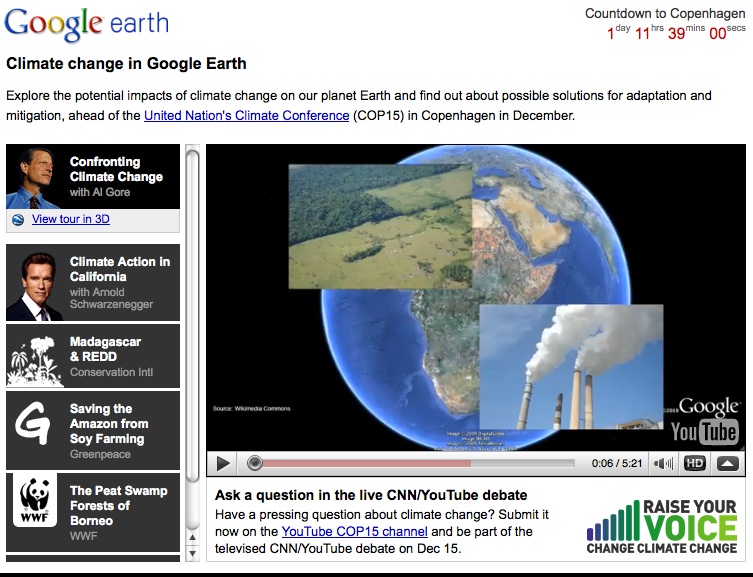This is a detailed screenshot of the Google Earth web page focused on climate change. In the upper left-hand corner, the page is branded with the Google Earth logo, featuring the iconic Google text in multiple colors: blue, red, yellow, and green. In the upper right corner, a countdown timer dramatically reads: "Countdown to Copenhagen: 1 day, 11 hours, 39 minutes, and 00 seconds."

The main header text at the top of the page states, "Climate Change in Google Earth," followed by a descriptive subheader: "Explore the potential impacts of climate change on our planet Earth and find out about possible solutions for adaptation and mitigation ahead of the United Nations Climate Conference (COP 15) in Copenhagen in December."

Running vertically down the left side of the page, five rectangular boxes present different climate change topics. These include:

1. "Confronting Climate Change with Al Gore"
2. "Climate Action in California with Arnold Schwarzenegger"
3. "Madagascar and REDD by Conservation International"
4. "Saving the Amazon from Soy Farming by Greenpeace"
5. "The Peat Swamp Forests of Borneo by WWF"

On the right side of the page, a YouTube video screen showcases an image of the Earth with overlaying square or rectangular photographs. The top photograph depicts an aerial view of green land, while the lower photograph features smokestacks emitting smoke towards the upper right.

At the bottom-right section of the page, there is a prompt for engagement: "Ask a Question in the Live CNN YouTube Debate. Have a pressing question about climate change? Submit it now on the YouTube COP 15 channel and be part of the televised CNN YouTube debate on December 15th." Beside this, in the far-right bottom corner, there appears a series of blue and green lines with the phrase "Raise Your Voice, Change Climate Change" promoting active participation.

This highly informative layout not only raises awareness about climate change but also encourages active involvement and discourse ahead of the significant UN Climate Conference.